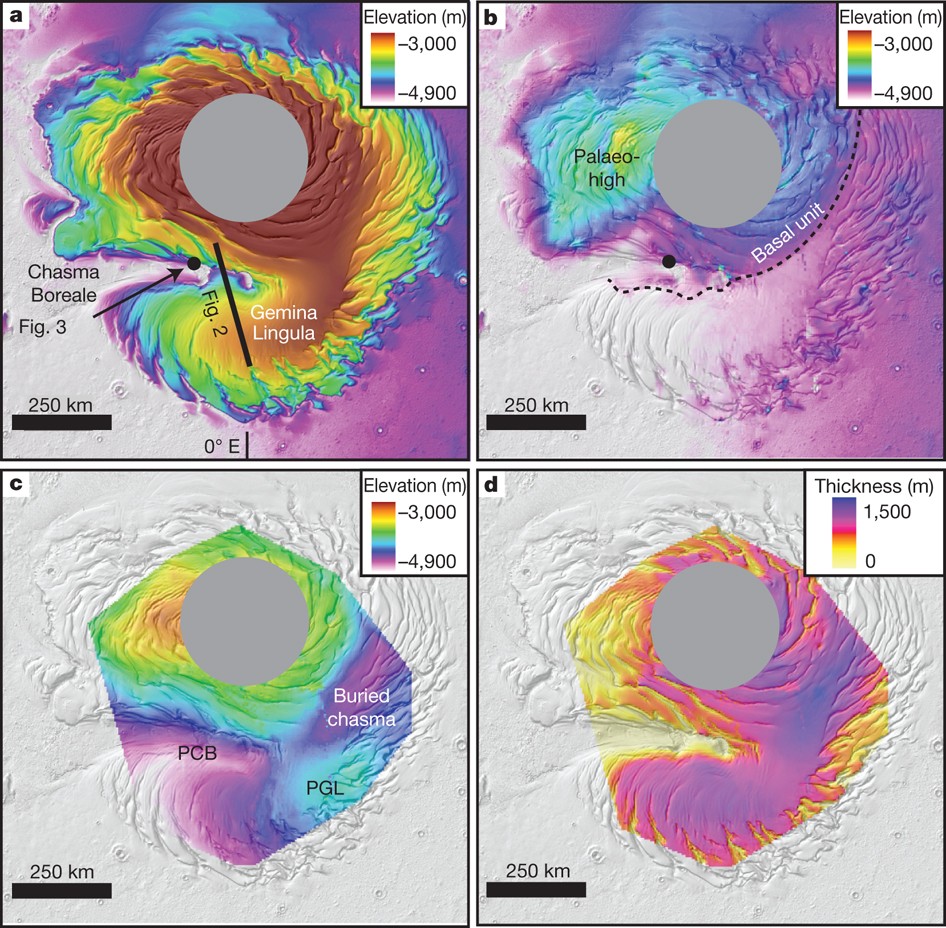The image comprises four colorful, labeled panels (A, B, C, and D) showcasing different aspects of elevation and thickness in a region potentially related to weather or geological analysis. Each panel features a color-coded scale for elevation or thickness with distinct labels and color gradients.

1. **Panel A (Top Left)**: Displays "Gemini Lingula Chasma Boreal, Figure 3" with an elevation range from -3000 to -4900 meters. The color gradient transitions from gray at the center to red, yellow, orange, green, blue, and purple. A scale marker indicating 250 kilometers is visible.

2. **Panel B (Top Right)**: Identically ranges in elevation from -3000 to -4900 meters. It includes labeled features such as "Paleo High" on the left and "Basal Unit" on the right, marked by a dotted line. The colors are primarily blues and purples, with fewer variations than Panel A.

3. **Panel C (Bottom Left)**: Also maintains the elevation range from -3000 to -4900 meters. It features "Buried Chasma," "PGL," and "PCB" among its labeled elements. The colors predominantly include greens, yellows, blues, and purples, presenting a different visual scheme than the other elevation panels.

4. **Panel D (Bottom Right)**: Distinctly labeled with "Thickness" instead of elevation, showing a scale from 15,000 to 0 meters. It uses a color gradient of yellows, purples, and pinks to depict thickness variations, and does not include specific labels for geographical features.

The panels are organized with A and B at the top, and C and D directly below them. The colors across all images are varied and include shades of gray, purple, blue, yellow, orange, green, and maroon, suggesting the data might be sourced from a radar system or a similar weather station program.